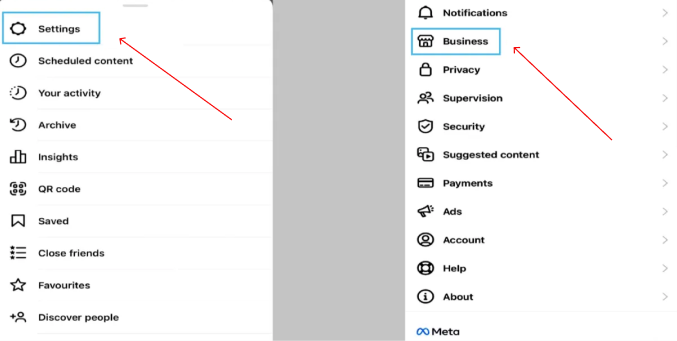The image predominantly features multiple columns filled with text and accompanying icons. 

On the far left side, there is a vertical column of icons, each followed by text explaining their purpose. The first icon is a gear symbol labeled "Settings," highlighted with a blue border around both the icon and the text. A red arrow points directly to this phrase, emphasizing its importance. Following the settings icon, there are icons for various categories including "Scheduled Content," "Your Activity," "Archive," "Insights," "QR Code," "Saved," "Close Friends," "Favorites," and "Discover People." 

In the center of the page, there is a plain gray column without any text or images, serving as a visual divider. 

To the right of this gray column is another set of icons, each explained by the adjacent text. The first icon in this right-hand column is a bell symbol labeled "Notifications." Below it is an icon of a store with the word "Business," framed by a blue border and indicated by a red arrow. Other icons in this column represent categories such as "Privacy," "Supervision," "Security," "Suggested Content," "Payments," "Ads," "Account," "Help," "About," and "Meta."

On the far right side of the page, each line includes small arrows pointing to the right, presumably indicating further navigation options for each line item.